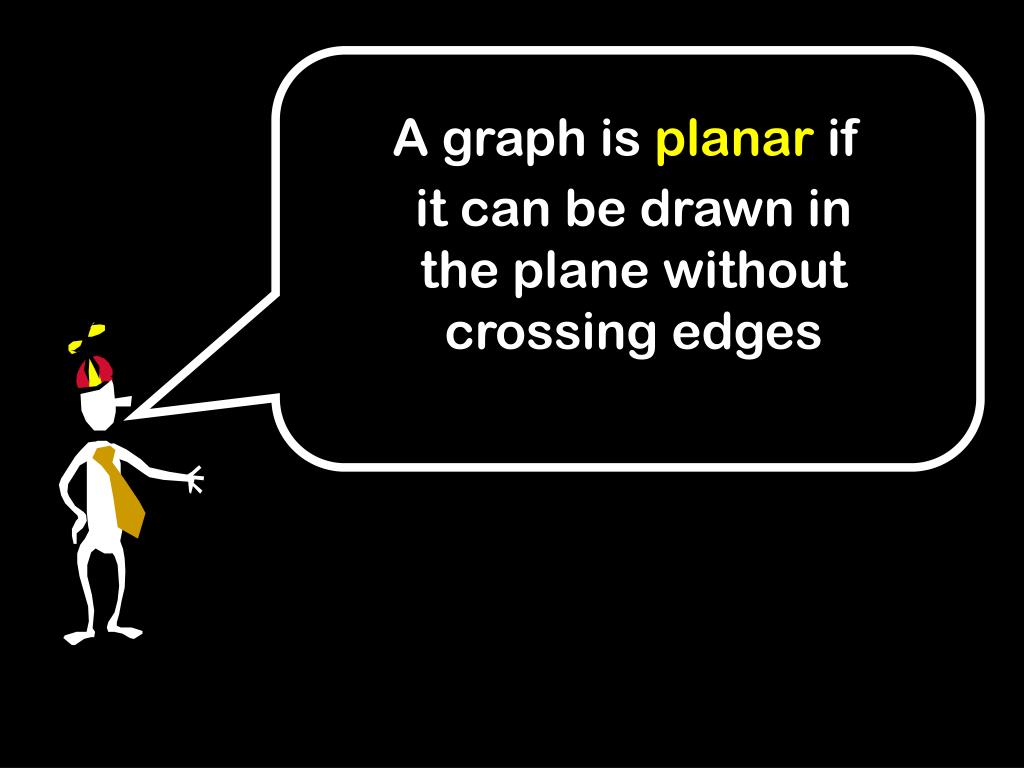The image features a minimalist, white stick figure with a distinct nose on an all-black background, positioned in the lower left corner. The figure is adorned with an orange tie and a red and yellow propeller hat. Extending towards the center of the image is a large, white speech bubble outlined in white, occupying much of the remaining space. Within the speech bubble, sans-serif text reads: "A graph is planar if it can be drawn in the plane without crossing edges." Notably, the word "planar" is highlighted in yellow, while the rest of the text remains white. This illustration, reminiscent of educational material, likely serves as a visual aid or reminder for a mathematical concept, presented in a clean, simple design.